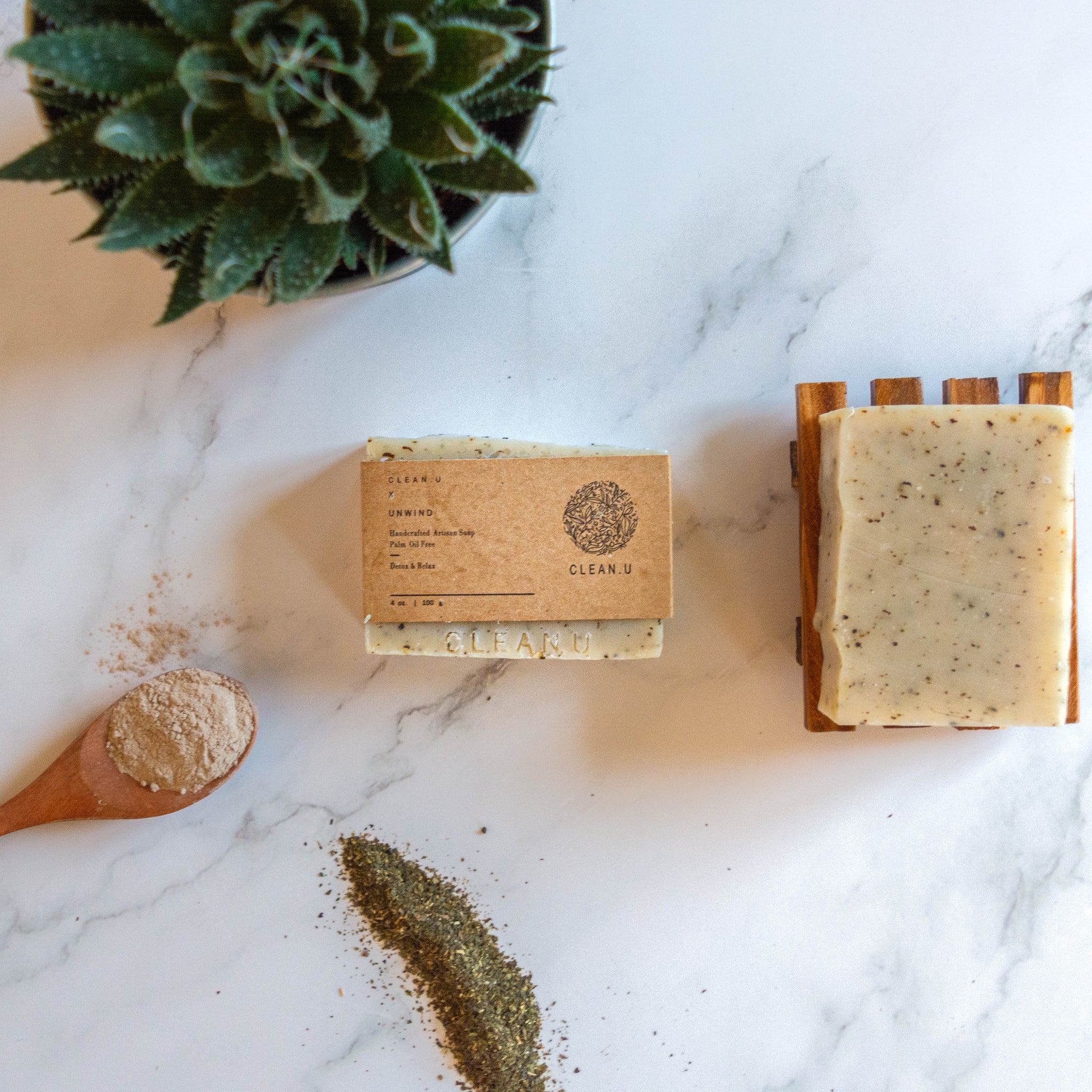The image is a detailed top-down view showcasing Clean U Natural Soap, placed on a white marble surface with gray veins. In the upper left-hand corner, there's a potted succulent plant with pointed, jagged, and bumpy leaves. The middle of the image prominently features a bar of soap wrapped in brown cardboard with the label "Clean U Unwind" and an indistinct logo resembling plant leaves. Adjacent to it, the same soap bar, displaying a tan color with green speckles, rests on a wooden soap dish. Below, a brown wooden spoon contains a beige powder with some spilled crumbs, and next to it lies an oval-shaped pile of a darker green powder, likely representing the soap ingredients. The composition and arrangement suggest a natural and organic theme, emphasizing the soap's handmade quality.